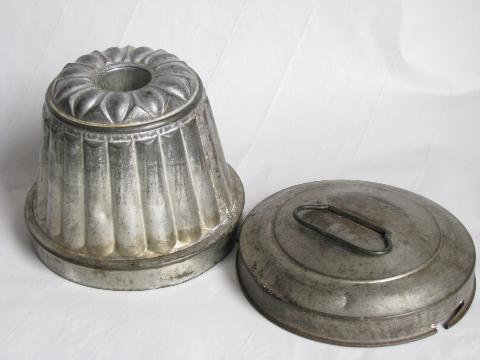The image features two aged metal objects positioned in a studio setting against a plain white background. On the left is an upside-down container, perhaps an antique Jell-O mold or flower pot, characterized by scalloped edges and a decorative patina. The molded item displays a band around its base, ridges resembling columns, and a top band featuring a leaf design, indicative of its frequent use and wear. The object also has a central hole and shows a gradient of discoloration from light to darker silvers. To the right of this container lies a metal lid, about the same size, reminiscent of an old-fashioned trash can lid. This lid is round, with a discolored finish in browns and grays, and is equipped with a metal handle in its center. The soft, diffused studio lighting, likely from a light box, creates a shadowless environment, and there is a slight wrinkling visible in the white background fabric or paper.